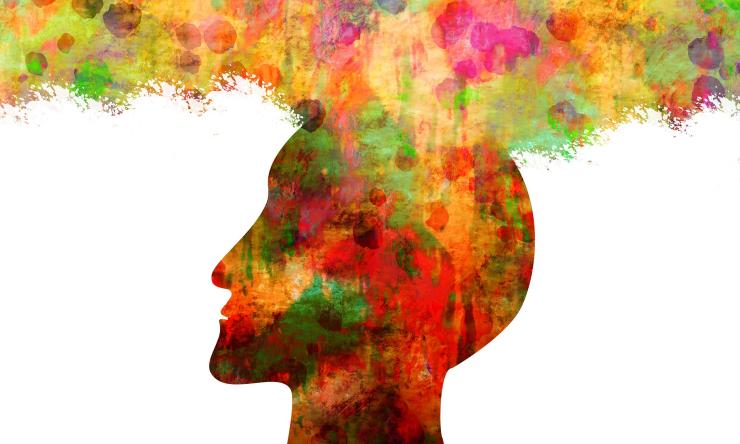The image depicts the silhouette of a gentleman's profile facing left, meticulously highlighting defining features like his nose, slightly open mouth, and bald head. The backdrop is a stark white, which accentuates the vivid explosion of colors emanating from the top of his head. These colors, resembling watercolor splatters or bushy, vibrant foliage, span a mesmerizing spectrum from greens, oranges, and reds to purples, blues, pinks, and yellows, with occasional delicate specks of black. While inside the silhouette, deeper shades of reds dominate, interspersed with touches of green and yellow. The overall impression is of a dynamic cascade of thoughts or creative energy erupting from the man's mind, transforming the minimalist silhouette into a rich tapestry of colors.